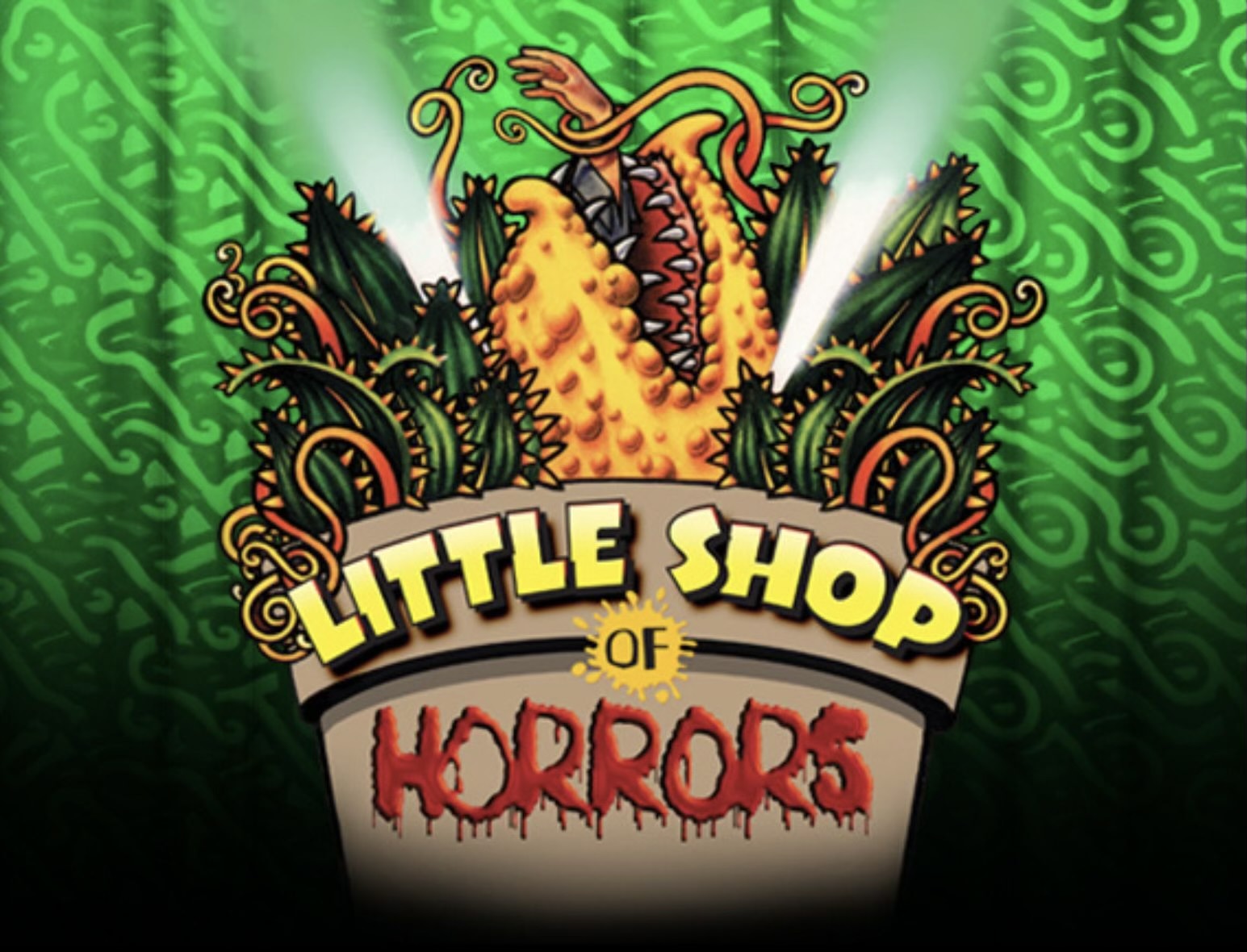The image appears to be an artistic rendering or title card for the movie "Little Shop of Horrors." The background is light neon green with tribal-like squiggly lines, creating a textured effect. At the base of the image is a black section from which a light tan flower pot emerges. 

The title text appears on the pot in a layered configuration: "Little Shop" is written in bold yellow letters at the top, "Of" is positioned in the middle within an orange splatter, and "Horrors" is at the bottom in red, dripping letters resembling blood. This gives the movie title "Little Shop of Horrors" a striking visual impact.

From the pot springs a collection of thorny, cactus-like plants with green leaves and sharp spiky stems that are red and yellow. Dominating the center of this chaotic growth is a monstrous, yellow-orange Venus flytrap-like plant with a gaping mouth full of sharp silver teeth and red gums. The plant appears to be in the act of consuming a person, with only an arm visibly sticking out of its mouth. One of the plant's tentacle-like vines is wrapped around the wrist of the arm, enhancing the horror theme. Additionally, two spotlights angle towards the plant from the left and right, drawing attention to the menacing scene.